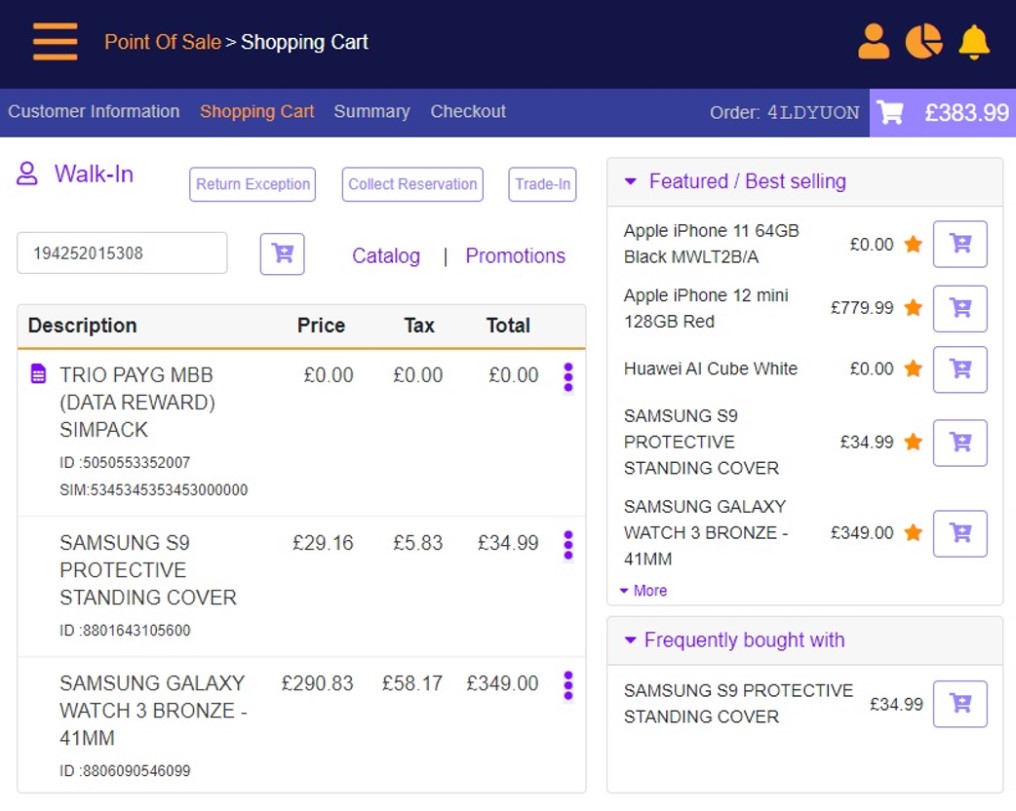Screenshot of a Point of Sale Shopping Cart for a computer equipment store, featuring a detailed interface. 

The top banner prominently displays "Point of Sale Shopping Cart." Below it, a blue navigation bar offers menus such as Customer Information, Shopping Cart Summary, and Checkout. To the right of this bar, there is a shopping cart icon showing a total price of £383.99.

On the left side of the screen, a detailed list of purchased items is visible, complete with descriptions, prices, tax, and totals. The items include:
1. Trio PAY-G MBB Data Reward SimPack
2. Samsung S9 Protective Standing Cover
3. Samsung Galaxy Watch 3 Bronze 41mm

The right side of the screen showcases featured and best-selling items available for purchase. Additionally, there is a drop-down menu titled "Frequently Bought With," which suggests the Samsung S9 Protective Standing Cover.